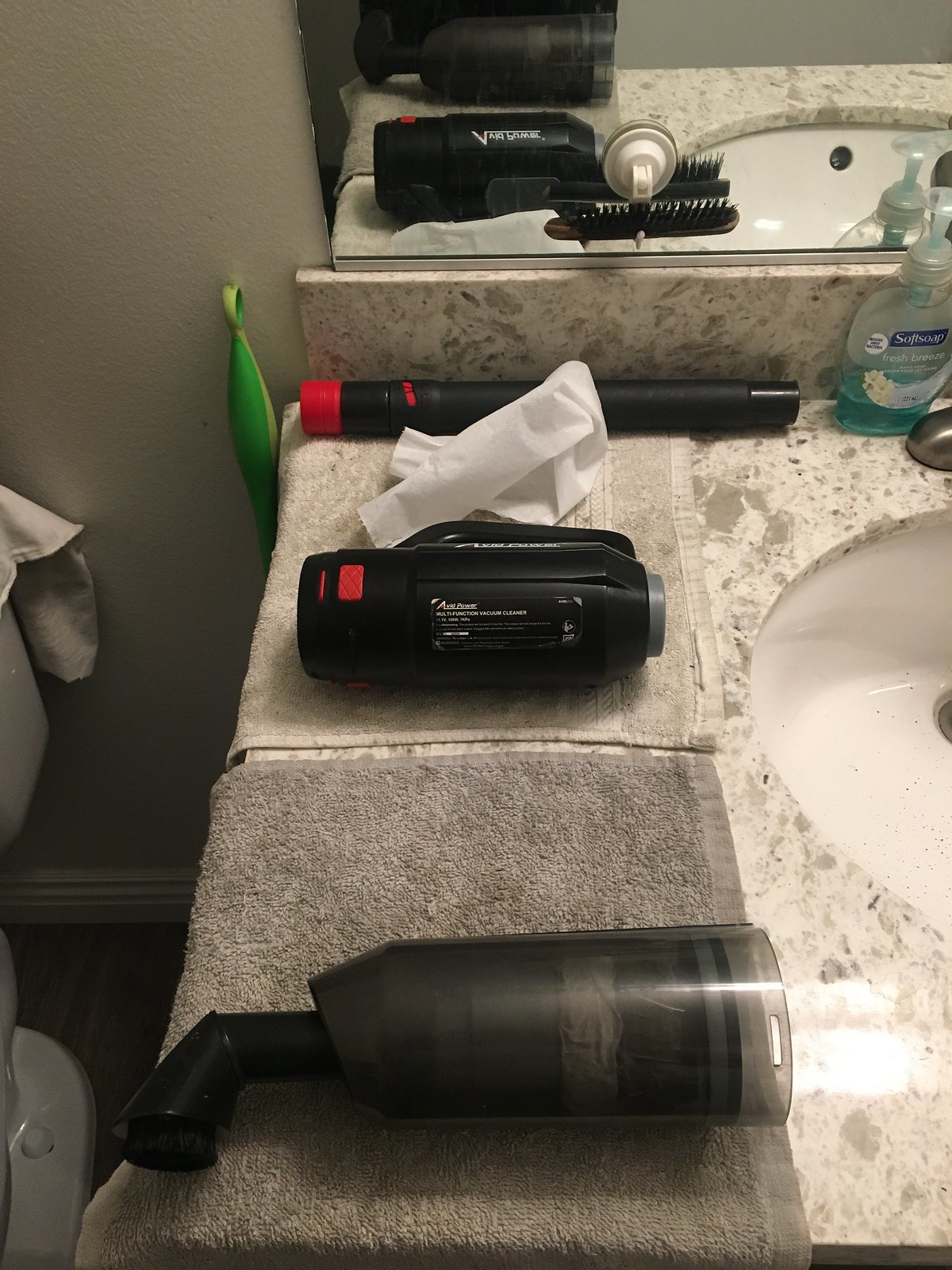This detailed image captures a bathroom scene, focusing on a light-colored, granite vanity countertop with white and gray marbling. A white ceramic sink with black hair specks is positioned on the right. On the countertop, there are two gray towels, and atop them lie a camcorder and various hair care products. A soft soap bottle, containing blue liquid and about three-quarters empty, sits near the sink. Part of a mirror with a suction cup hook is visible above the vanity's backsplash. A black dryer with a wand and brush attachment, along with a Swiffer brush, are also seen. Alongside the vanity, a partial view of the toilet with a rag draped over its back is noticeable. The bathroom features a gray-colored wall in the background. In the foreground, a peculiar gray cylinder with a bent black tube is lying on a towel, adding a mysterious element to the scene.